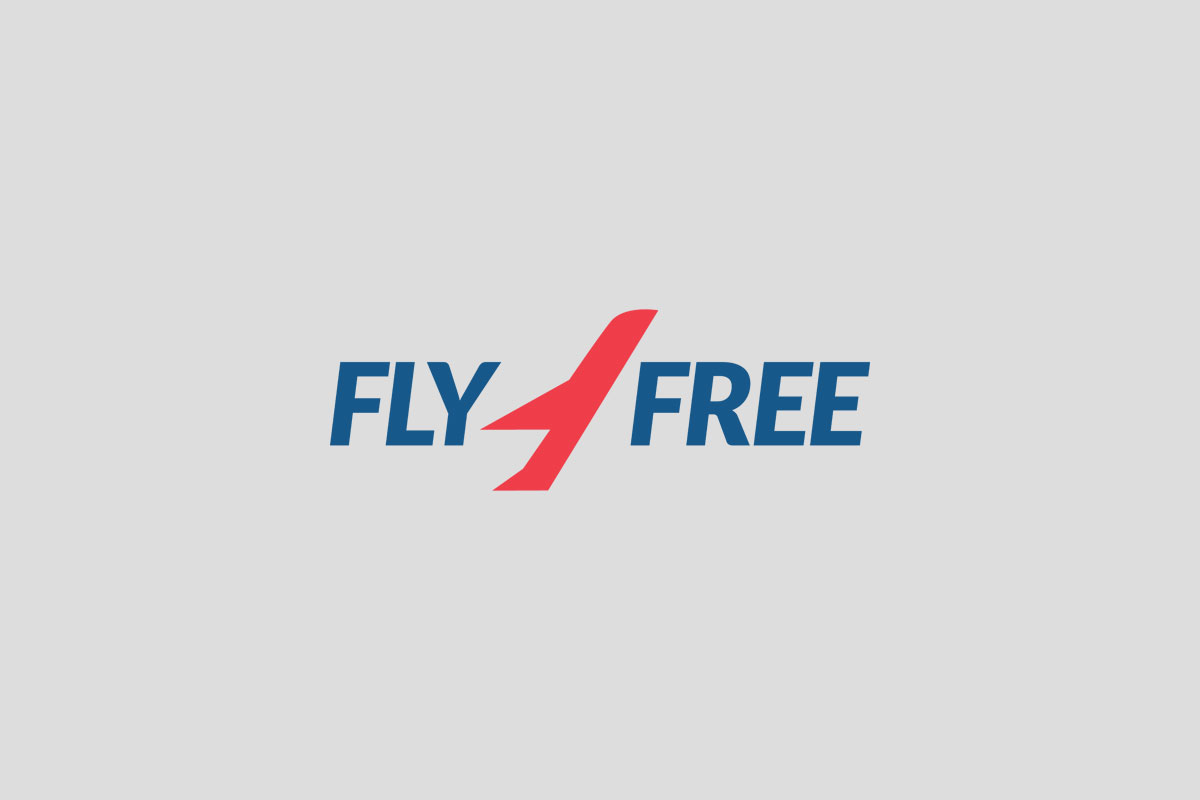**FlyFree Logo Imagery Detailed Description**

This is the logo for FlyFree, an entity presumably dedicated to travel services. The logo features the word "Fly" followed by a stylized, small jet airplane icon aiming upwards, symbolizing flight and adventure. The jet is placed between "Fly" and "Free," seemingly propelling upwards towards the free skies, which are depicted in a vibrant red color, signifying energy and excitement. Although the exact services offered by FlyFree are not explicitly known, the imagery suggests it might be a travel service provider, likely offering deals on flights, accommodations, and travel planning. The accompanying website is assumed to be flyfree.com, where users might find resources such as affordable flight tickets, hotel bookings, travel destination guides, news, and blogs related to the travel industry. The logo projects a sense of freedom and exploration, integral elements of the travel experience.